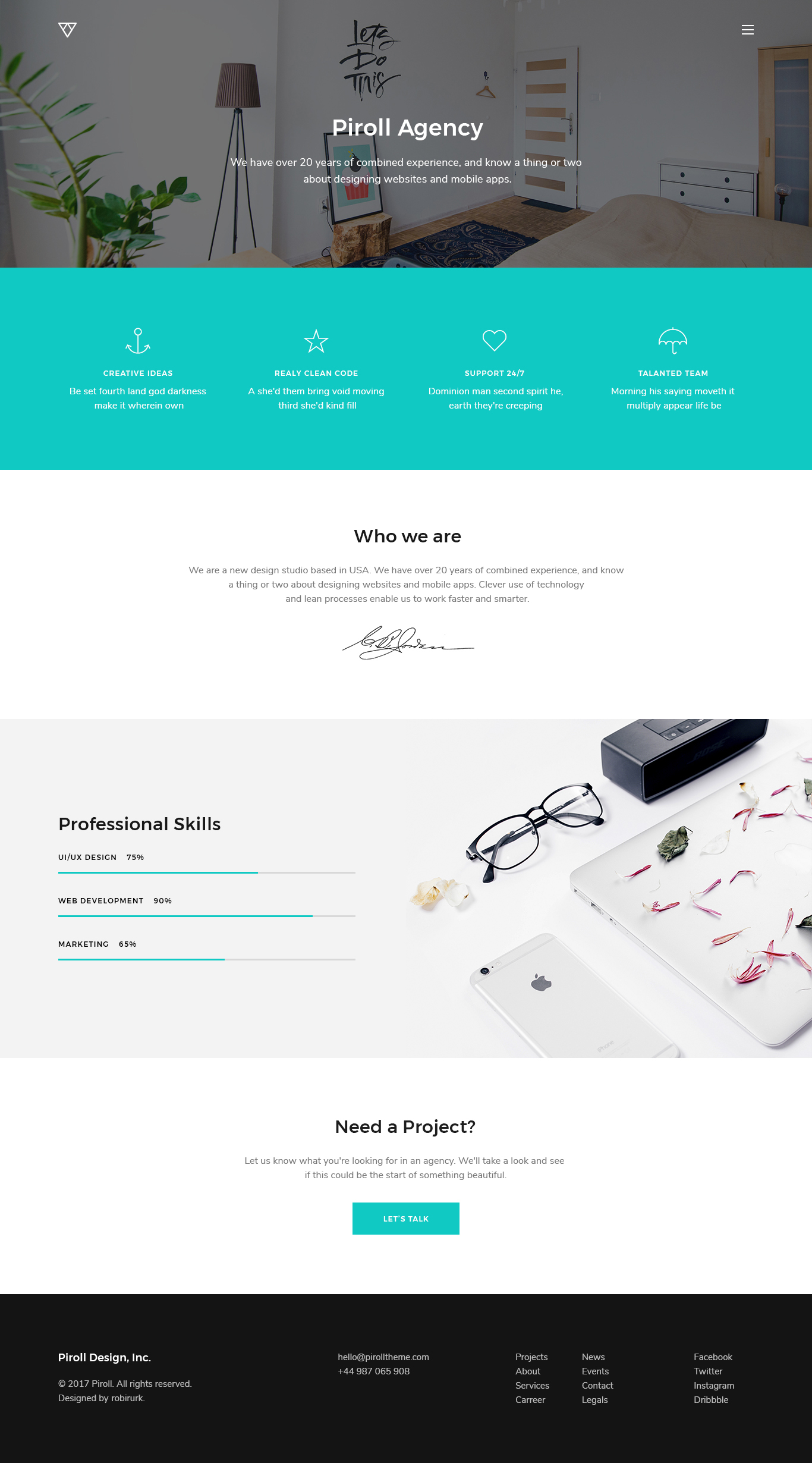This photo captures the homepage of a payroll agency's website, which features a clean and modern color scheme dominated by shades of turquoise and white. The website's name is prominently displayed in white font overlaying a high-resolution image of a contemporary bedroom. The bedroom, characterized by its modern aesthetic, boasts white walls and pale wood flooring. At the room's center is a large bed covered with a beige blanket. Below the title, there is text in a very small font that is difficult to read. 

The room is tastefully decorated with several green potted plants that add a pop of color. There's a square, dark blue rug on the floor, enhancing the room's chic vibe. A black, cursive inscription is elegantly scripted on the wall, adding a touch of personality. An eye-catching piece of art, framed in black, features an abstract design in blue, red, and black hues. Completing the room's decor is a dresser with several drawers, each equipped with two knobs. This impeccably styled room exudes a serene and organized atmosphere, setting a sophisticated backdrop for the payroll agency's online presence.